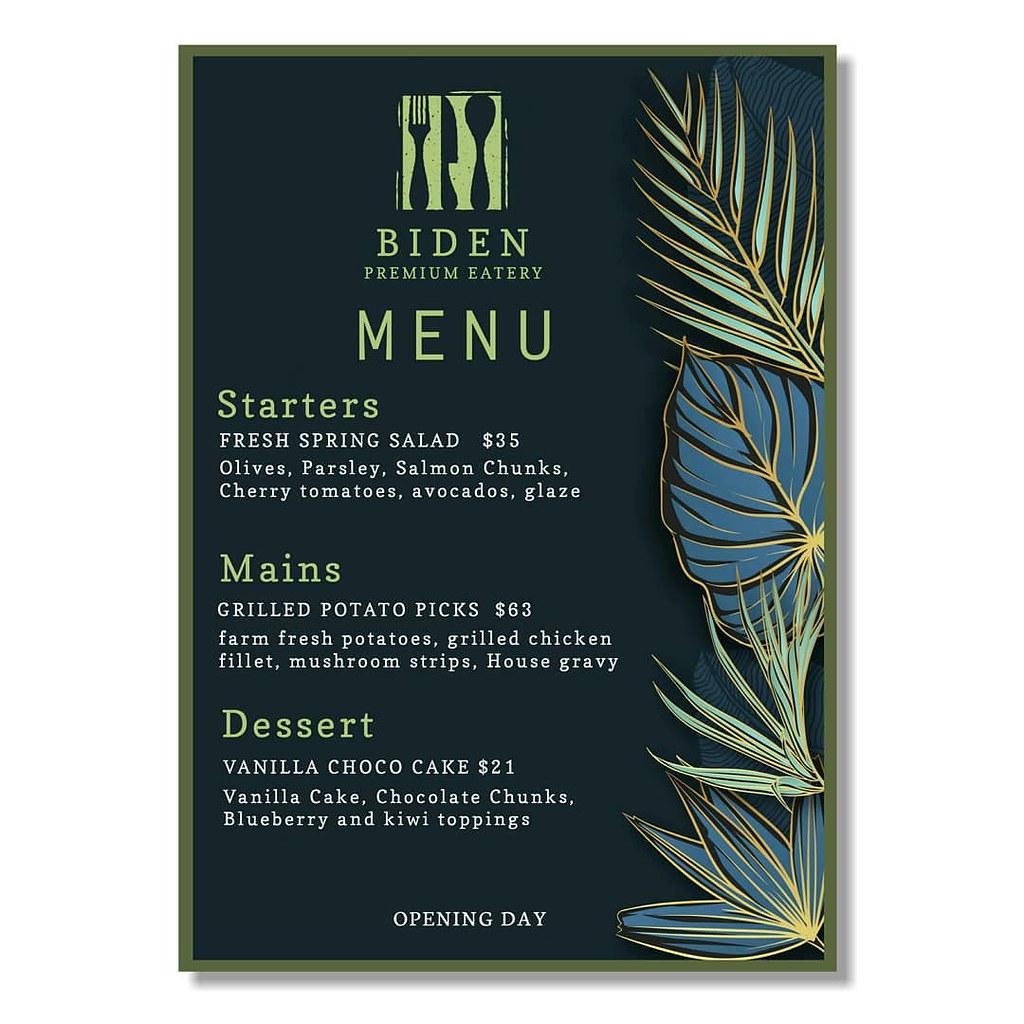The image depicts a detailed graphic menu for Biden Premium Eatery. It has a vertically oriented rectangle with a very dark green background, framed by a narrow olive green border. At the top center, there is a logo featuring a green square with a fork, knife, and spoon positioned from left to right. Below the logo, in light green text, the words "Biden Premium Eatery" are prominently displayed, followed by the word "MENU" in the largest sans serif font.

On the right side of the design, there are artistically drawn tropical plants and leaves. These include a thin-bladed leaf at the top, a larger blue leaf below it, and even longer, strand-like leaves followed by a green leaf that combines characteristics of both broad and strand-like leaves.

The menu content is split into three sections: Starters, Mains, and Dessert, each title displayed in light green uppercase text. The text for each dish within the sections is white. 

- **Starters:** Fresh Spring Salad, $35 featuring olives, parsley, salmon chunks, cherry tomatoes, and avocado glaze.
- **Mains:** Grilled Potato Picks, $63 with farm-fresh potatoes, grilled chicken filet, mushroom strips, and house gravy.
- **Desserts:** Vanilla Choco Cake, $21 composed of vanilla cake, chocolate chunks, and blueberry and kiwi toppings.

Centered at the bottom of the menu in white capitalized text are the words "OPENING DAY".